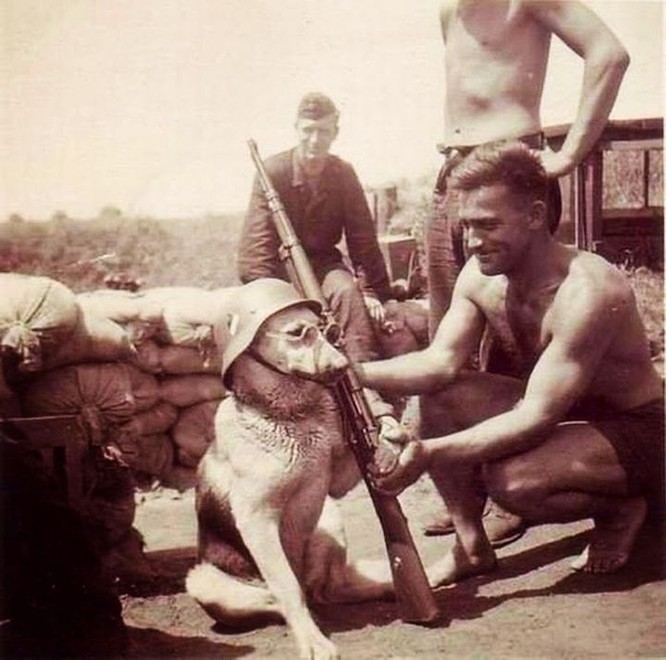The black-and-white photograph captures a World War II setting with three soldiers and a dog at what appears to be a military base camp. The scene is fortified with sandbags, suggesting a wartime environment. Central to the image is a German Shepherd dressed comically in military gear, including round-rimmed sunglasses and a helmet strapped to its head. The dog, which has light-colored fur with darker facial spots, is positioned to look like it is shouldering a rifle. One soldier, crouching and wearing only shorts, holds the dog's paw and helps prop up the rifle with a wooden stock. Another shirtless soldier stands behind him, and a third fully-dressed soldier with a military cap is seated on the sandbags, smiling. In the background, there appears to be a jeep or shed, indicated by visible windows, and low shrubbery stretches out to the horizon, hinting at a warm, possibly Pacific Theater location during the war.